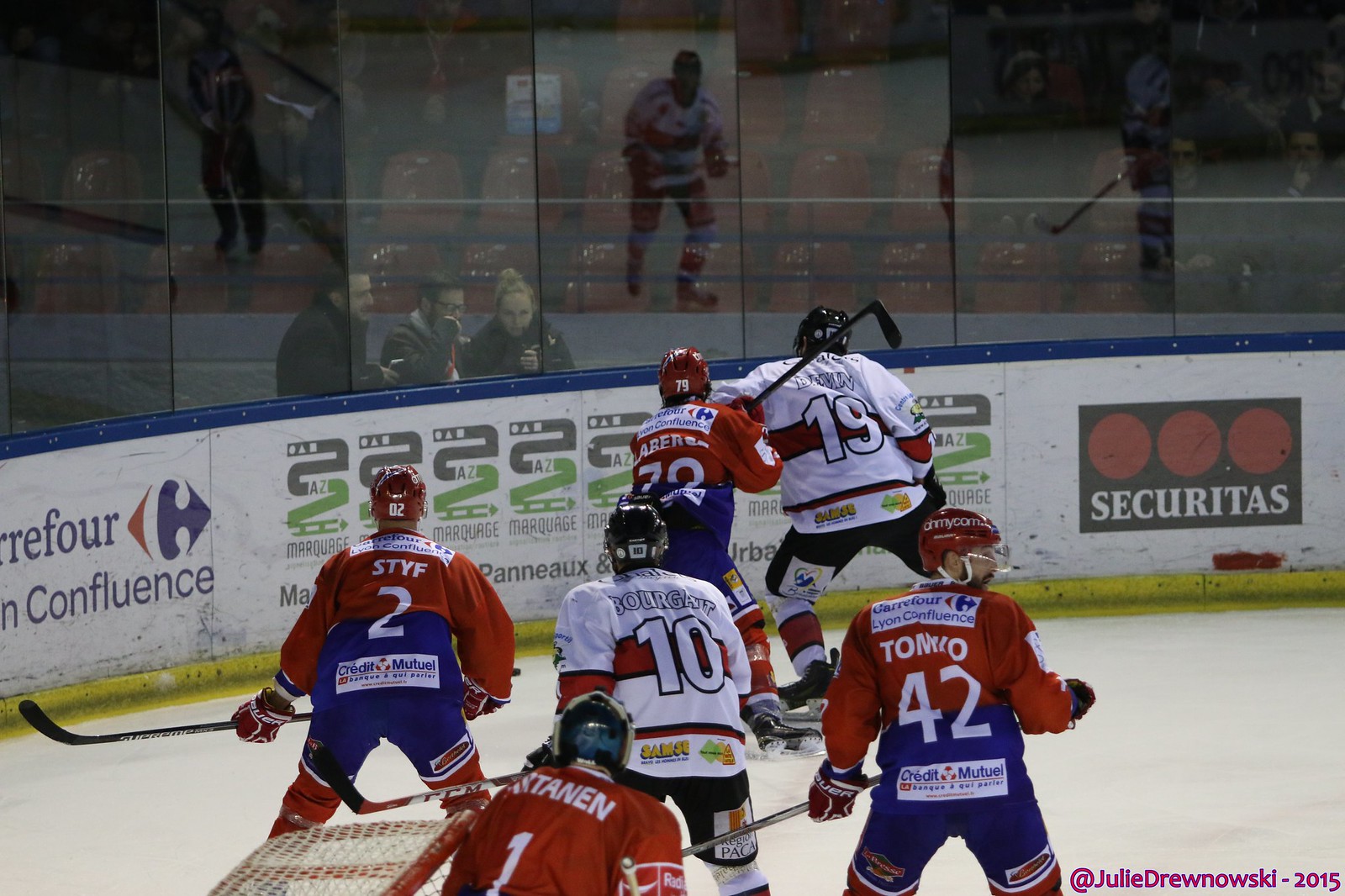The image captures the action of an ice hockey game with six players on the ice, their backs mostly facing us. Four of the players are wearing red and blue jerseys: number 2 (Stief), number 79, number 1 (Stannon), and number 42. The opposing team consists of two players in white jerseys with numbers 10 and 19. The scene appears to be a practice round, as the stadium seats in the background are mostly empty, save for a few spectators. Notably, three people—a woman and two men in coats—stand close to the rink, possibly coaches or medical staff watching intently.

The rink’s sidewall is adorned with several advertisements on a white background, featuring names such as Securitas, Panneaux, and Confluence. The bottom of the wall has a yellow border, topped with blue. The reflection on the class above reveals a few more spectators seated further back, adding depth to the scene.